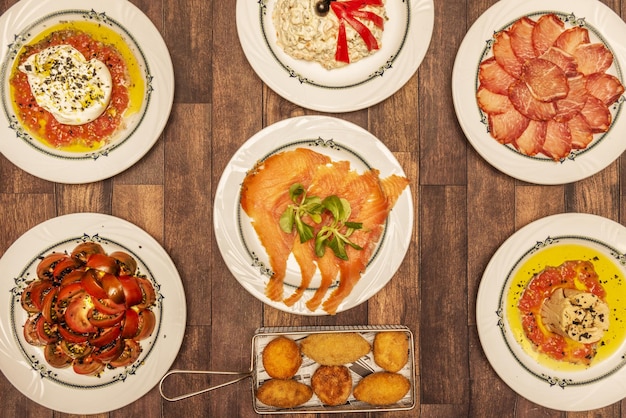In this detailed aerial shot of a rustic wooden table, we see a delightful assortment of dishes, each served on a white plate, capturing a diverse culinary spread. At the center of the table, surrounded by greenery, is a dish featuring succulent salmon paired with vegetables. To the left, a plate overflowing with savory seasoned tomatoes catches the eye. Adjacent to it is an egg-based dish, possibly an omelet, decorated with a rich mixture of seasoned yolk and tomatoes. Below the salmon, a hearty platter showcases strips of crispy bacon or ham, adding a meaty contrast to the meal. A uniquely arranged dish, which might be an omelet or rice, is distinguished by its medley of ingredients including seasoned egg and tomato. Completing the array is a cylindrical white food item garnished with a colorful red and yellow sauce, and a metal basket at the bottom center, brimming with golden fried items. Each dish, from the appetizing soups to the basket of fried fish, presents a feast for the eyes and promises a delightful dining experience.